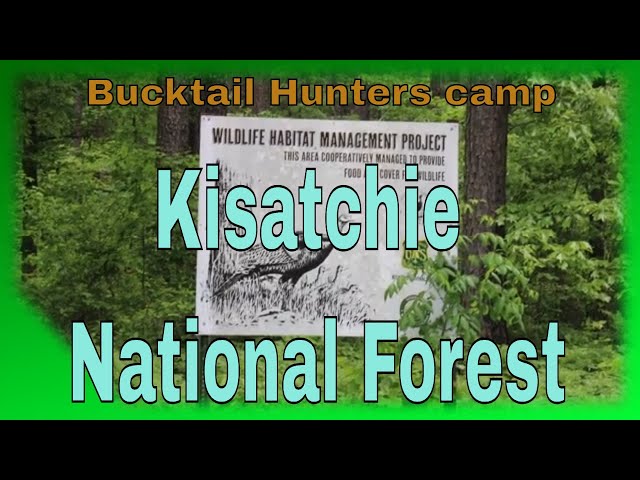The image appears to be from a slide presentation about the Bucktail Hunters Camp in the Kisatchie National Forest. At the top of the image, the title "Bucktail Hunters Camp" is prominently displayed in orange text. Across the middle of the image in large, light blue letters outlined in black, it reads "Kisatchie National Forest." The picture itself is bordered by a vibrant green fade-out. 

The central focus of the photograph is a dense wooded area filled with trees and lush vegetation, suggesting a healthy forest ecosystem. In the midst of the forest, a black and white sign stands out, displaying the words "Wildlife Habitat Management Project" along with the message, "This area cooperatively managed to provide food and cover for wildlife." A drawn image of a pheasant or peacock is visible on the bottom left of the sign. The setting depicts a peaceful nature preserve, emphasized by the rich greenery and the detailed brush surrounding the area.